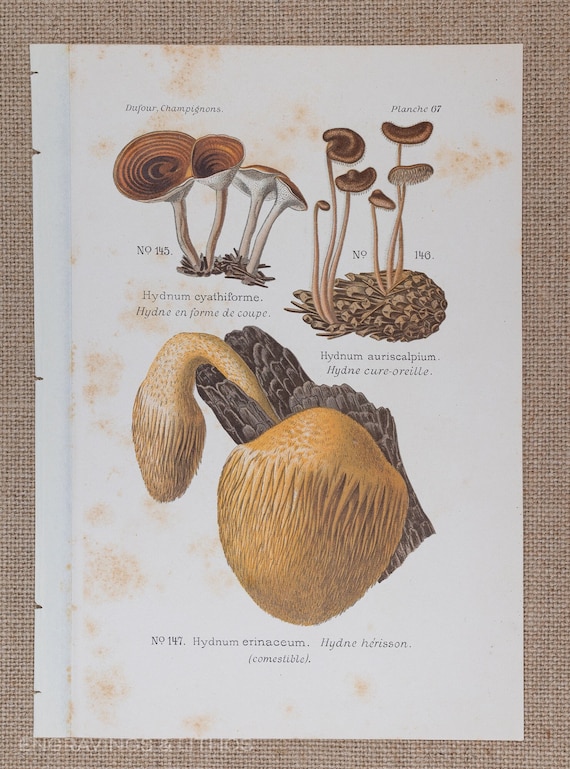The image appears to be an illustration of various types of mushrooms and fungi, displayed on a white paper background with a tan, stitched cloth border. In the upper left section, there are several white-stemmed mushrooms with spiraling brown caps labeled "Dufour champignons" and "No. 145, Hydnum chiathiform." Adjacent to them, on the top right, are thin-stemmed mushrooms with brown tops resembling pine cones, marked "No. 146, Hydnum oroscalpium." The bottom middle features a yellowish mushroom-like growth that appears fleshy and coral-like at the base, identified as "No. 147, Hydnum arenicum." Various parts of the illustration contain scientific names and associated numbers, adding to its botanical and mycological specificity.